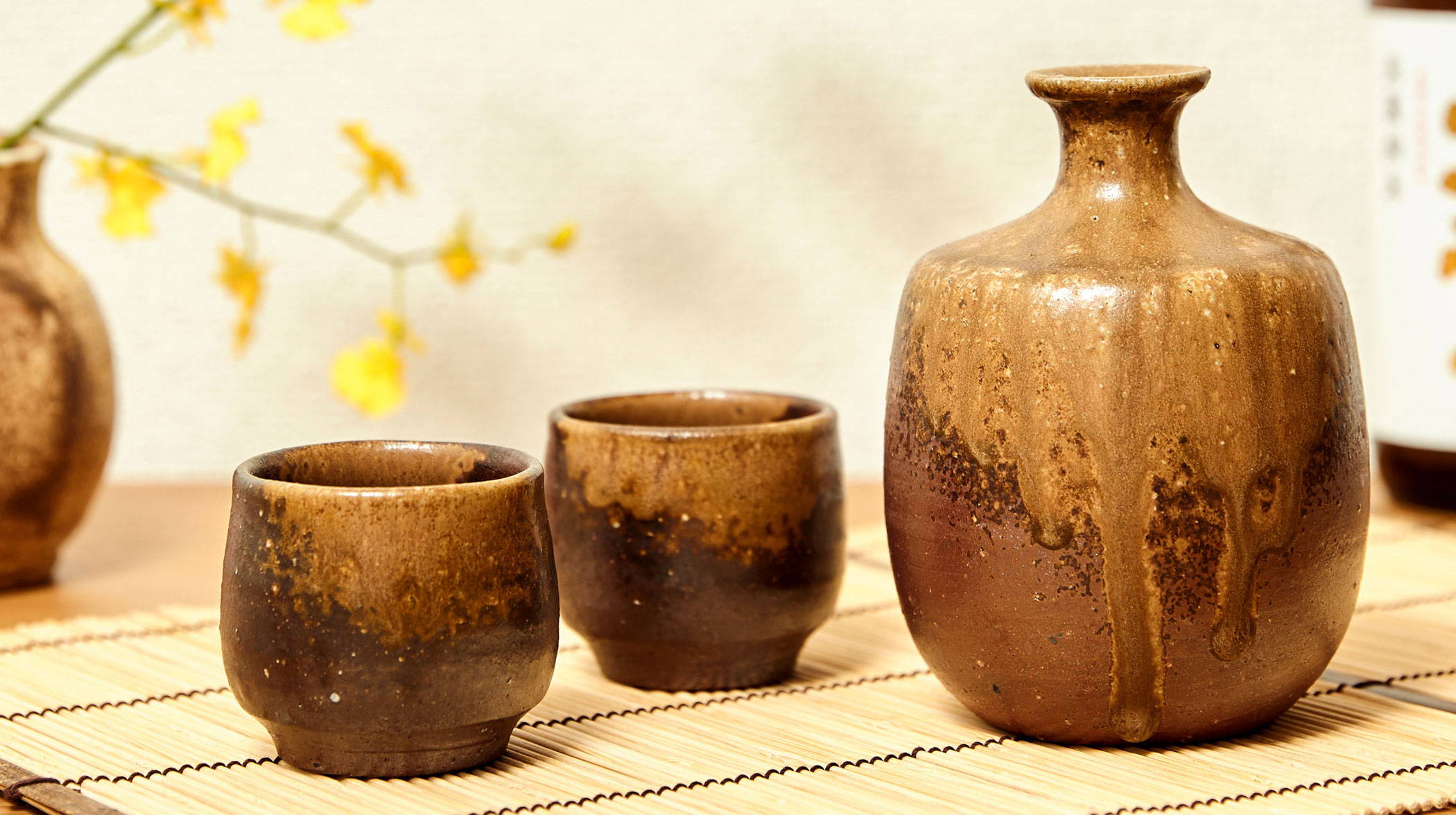In the image, three artisanal brown pottery items are thoughtfully arranged on a light-colored bamboo placemat that features subtle thin black stripes running across it. On the left, there are two squat, handleless glasses with wide openings at the top and slightly narrower bases, reflecting a handcrafted, old-timey charm with their varied shades of brown. To the right, positioned between the glasses and the edge of the mat, is a narrow-mouthed jug with a wide base, designed perhaps to hold water or other liquids. Surrounding the pottery is a tastefully styled setting: to the left, in a wooden vase, thin branches adorned with vibrant orange-yellow leaves add a touch of nature's elegance, while the background features an off-white wall, partially blurred, that holds an ambiguous bottle with a white label on the right side. The overall scene evokes a serene, rustic aesthetic, reminiscent of traditional craftsmanship and warm, earthy tones.